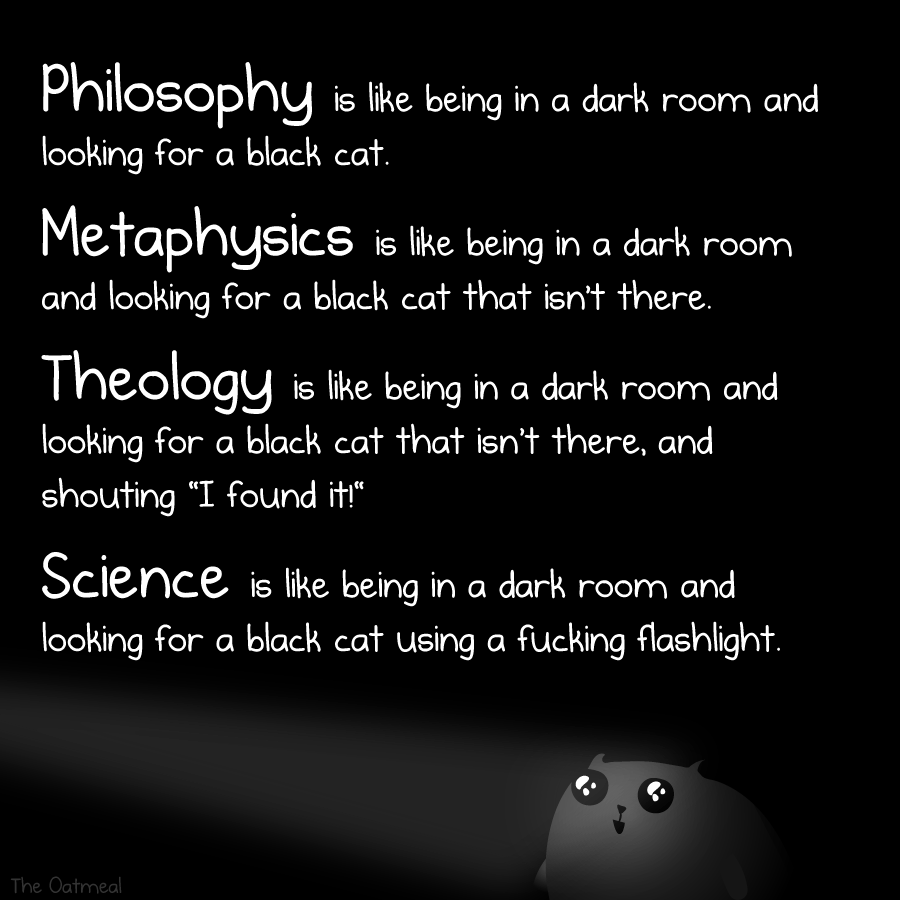The image features a predominantly black background, with a thought-provoking text in white letters occupying most of the space. Created by an artist known as Oatmeal, the text humorously delves into philosophical concepts: "Philosophy is like being in a dark room and looking for a black cat. Metaphysics is like being in a dark room and looking for a black cat that isn't there. Theology is like being in a dark room and looking for a black cat that isn't there, and shouting, 'I found it.' Science is like being in a dark room and looking for a black cat using a fucking flashlight." In the bottom right corner, a small grey cartoon kitten with large, glossy eyes and an open smile looks up at the text as though engaged by it. A gradient shines a subtle beam of light on the kitten's face. The artist's name, 'the oatmeal,' is subtly placed in gray in the bottom left corner.